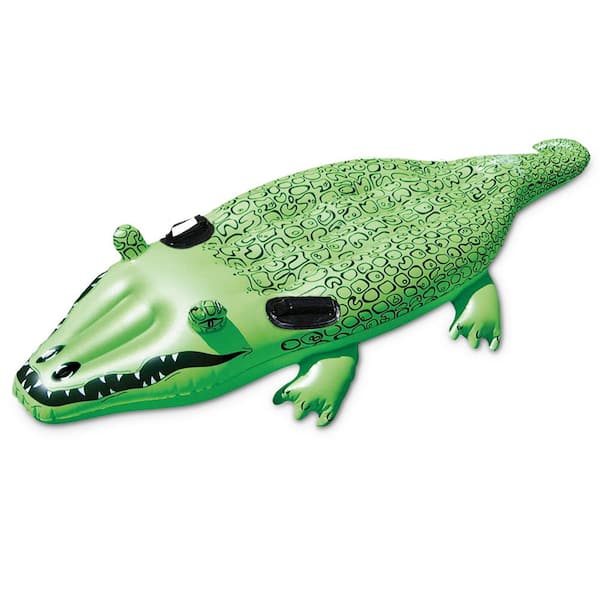The image showcases a single inflatable pool toy designed in the shape of a cartoon-like, lime-green crocodile. The background is entirely white, placing full emphasis on the elaborate details of the floatation device. This crocodile inflatable features a wide-open, graphically designed mouth complete with visible teeth, and a pair of nostrils on its snout. The eyes are prominently protruding, giving it an animated appearance, while the stubby feet with three toes each add a charming touch. The back of the inflatable is adorned with a varied pattern of circles, ovals, and squares to mimic the scales of an actual crocodile. Black patches located behind the eyes serve as handles, providing stability for a child or person who wishes to lie or sit atop it while floating. Overall, the inflatable crocodile is substantial in size, making it suitable for a child to comfortably stay on, blending playful aesthetics with functional design.